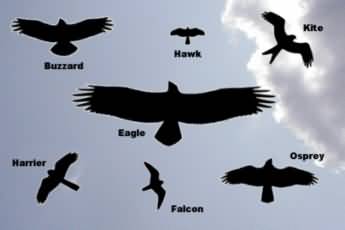The image depicts black silhouettes of various bird species against a grayish-blue sky with wisps of white clouds. There are seven birds in total, outlined and filled uniformly in black, with their wings fully outstretched as if seen from below. At the very center is an eagle, the largest bird in the picture, showcasing expansive wings with finger-like tips. Surrounding the eagle, arranged clockwise from the top left, are different species: starting with the buzzard, identifiable by its wide wings with distinct finger-like projections; followed by the hawk in the top center, the smallest bird with notably long wings; the kite in the top right, with curved wings and a distinctive tail resembling a mouse cursor; the osprey in the bottom right, characterized by medium-sized wings and pointed tips; the falcon in the bottom center, with long, pointed wings and a small tail; and lastly, the harrier in the bottom left, featuring elongated wings and a particularly pointed tail. The overall layout offers a comparative view of their varied shapes and sizes.